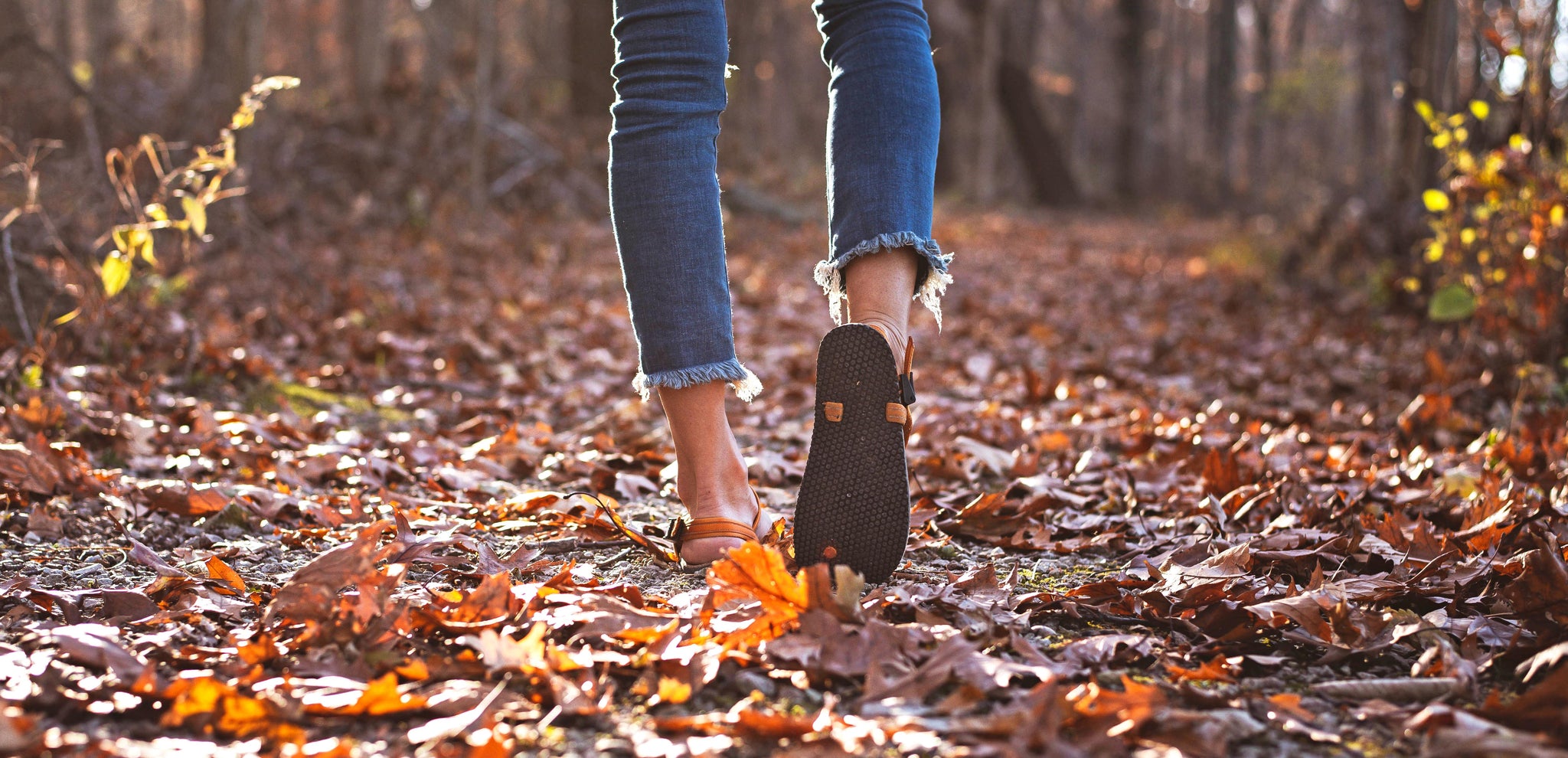In this image, we see the slender legs of a woman walking on a dirt trail blanketed with fallen autumn leaves, predominantly in shades of brown and orange, some appearing crusty and ready to break apart. The photograph captures just her legs from the knees down, adorned in frayed, cropped blue Levi's jeans that end at her ankles. She is wearing sandals with black bottoms and orange straps that wrap around the heel, resembling flip-flops with added support. The dirt path, illuminated by the warm, low-angle light of a sunrise or sunset, winds through a forest setting, with the sun casting its glow from the left of the image. The forest floor is rich with the colors of fall, while the trees on either side of the trail are just visible at their bases, their upper parts out of view or blurred, adding to the autumnal atmosphere. The woman's right foot is mid-step, showing the underside of her sandal, while the left foot is firmly planted on the ground. The scene is serene and picturesque, capturing a quiet, reflective moment in nature.